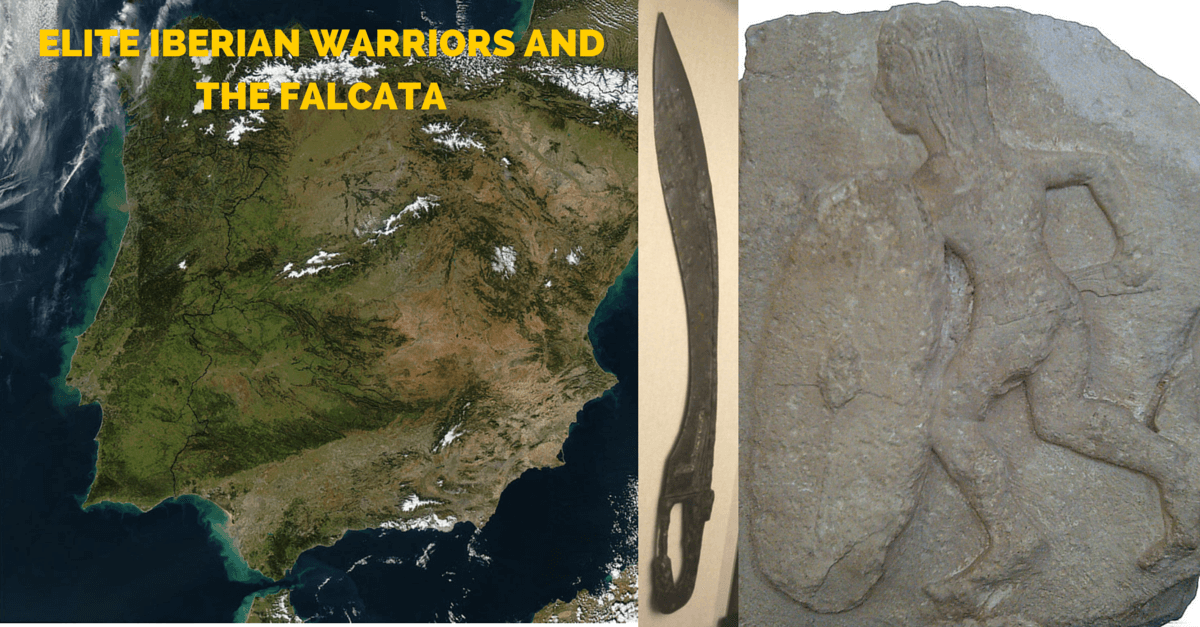The image is divided into three distinct segments. On the left, there is an aerial, almost satellite-like view of a landmass that appears to be an island or part of a peninsula, surrounded by water on at least three sides. This section is labeled with bold yellow text at the top, reading "Elite Iberian Warriors and the Falkata". In the middle segment, there is a thin, rectangular photograph of an ancient weapon. This weapon, identified as a Falkata, has a distinctive curved blade and a small handle at the bottom, reminiscent of a machete without a full grip. On the right segment, a stone carving depicts an ancient warrior. The carving, set in an off-white rock, shows a figure with long hair holding a large elliptical shield in the left hand and the Falkata in the right hand, poised as if in battle. The combination of these elements provides a historical snapshot highlighting the elite warriors of the Iberian Peninsula and their iconic weaponry.